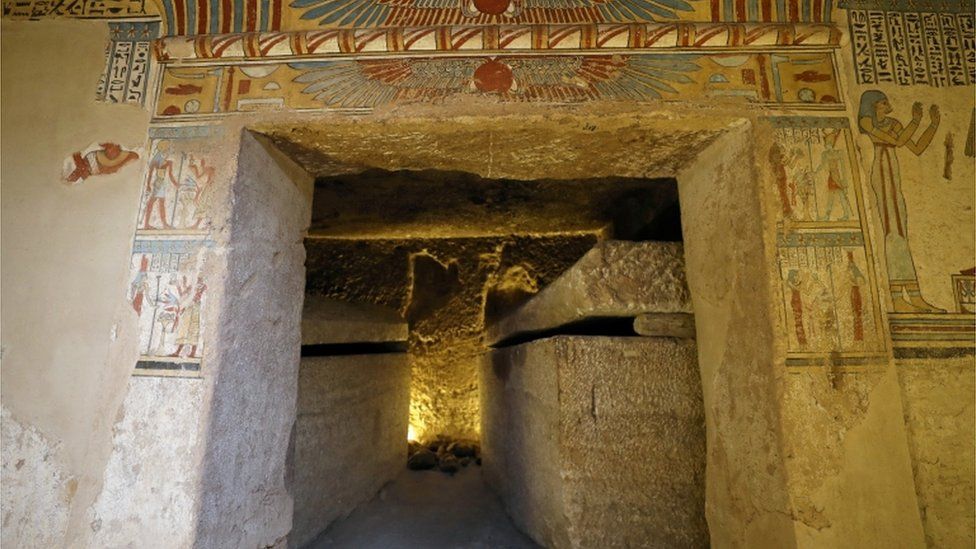This detailed image showcases the entrance to an ancient Egyptian pyramid, potentially leading either to the pyramid itself or a chamber within. The entrance is adorned with extensive hieroglyphics and traditional Egyptian imagery, featuring figures in traditional attire with raised and extended hands. Above the doorway, there is a prominent sun symbol reminiscent of the sun god Ra, encircled by an array of feathers, with another similar design situated above it, comprising a red central sun and predominantly blue feathers with some red accents.

The pyramid's tan stone walls contrast with the vibrant maroon, blue, and gold designs embellishing the entrance frame. Upon peering through the doorway, a corridor stretches back approximately 25 to 30 feet to a lit back wall, flanked on each side by rectangular stone containers—likely sarcophagi—with their lids in place. These prominent features within the corridor, combined with the rich decoration and hieroglyphics outside, vividly underscore the historical and cultural significance of this ancient site.